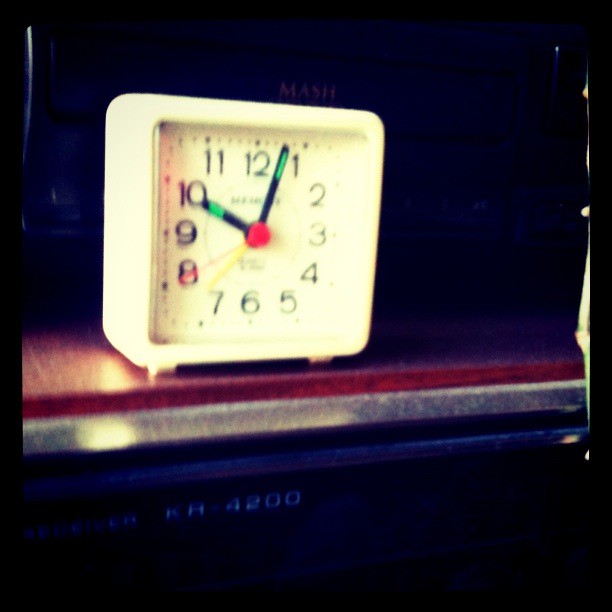This photograph features a small, square, off-white analog alarm clock reminiscent of the 1990s style. The clock face is adorned with black numerals and matching black hour and minute hands. These hands are accented with bright green neon paint, designed to glow in the dark for easy reading without needing external light. The second hand stands out in a striking red, as does the center of the dial. The clock rests on an indistinct table surface, captured against a backdrop that is dark and somewhat blurred, lending a slightly fuzzy appearance to the entire image. Despite this, the clock's design and function remain clearly discernible.